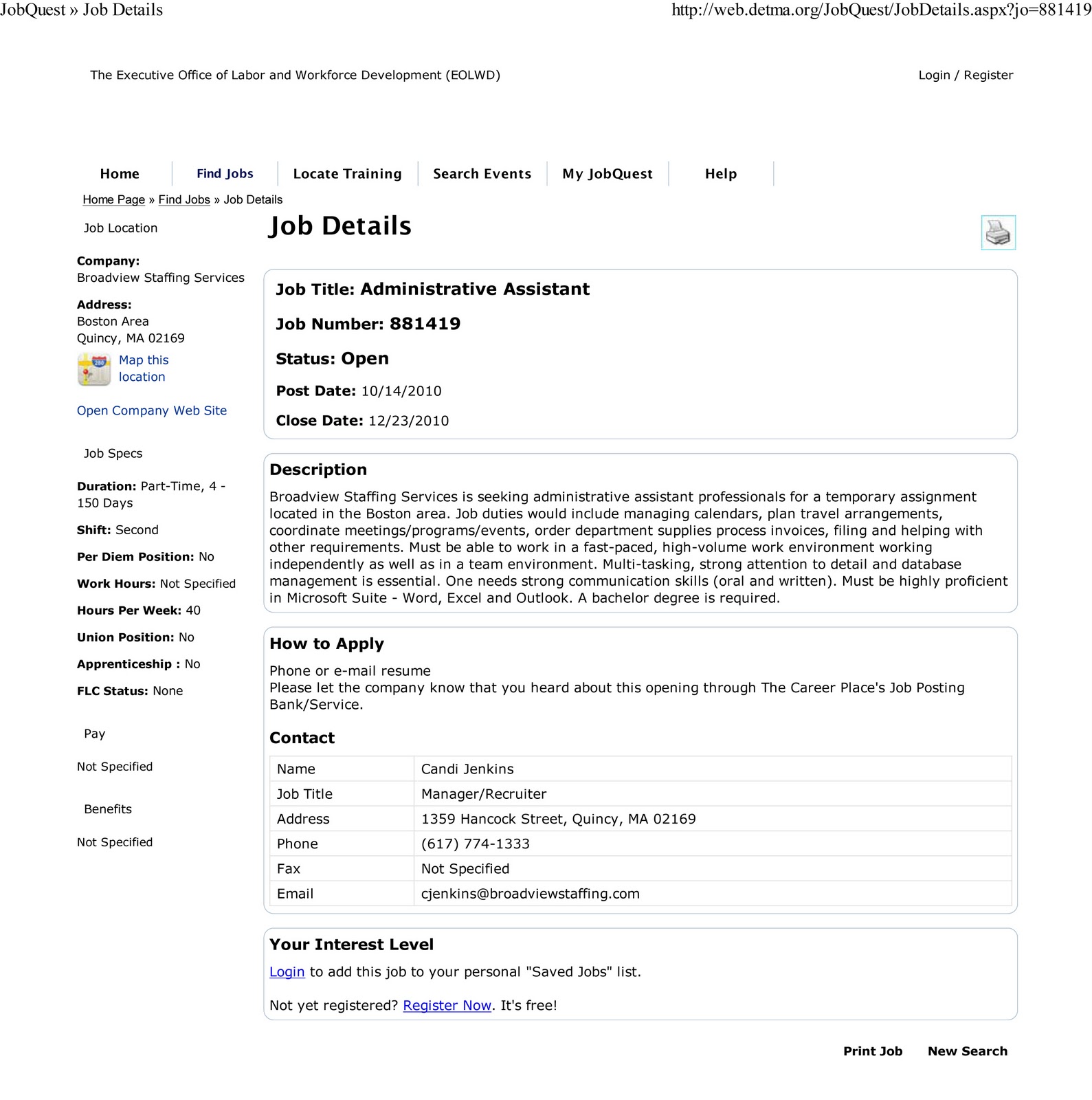The image displays a screenshot of a job search site known as web.detma.org. It showcases a detailed job listing for the position of an Administrative Assistant, which is currently open. The job description provides comprehensive details about the role and instructions on how to apply, including contact information and an associated email address. The site features a navigational menu at the top with various sections such as "Homepage," "Find Jobs," "Job Details," "Locate Training," "Search Events," "My Job Quest," and a "Help" section. The job listings on this site are informative, indicating whether the position is part-time or full-time, details on shift work, required weekly hours, union status, apprenticeship opportunities, and FLC status. Additionally, essential information such as pay, benefits, and other relevant factors are clearly outlined.